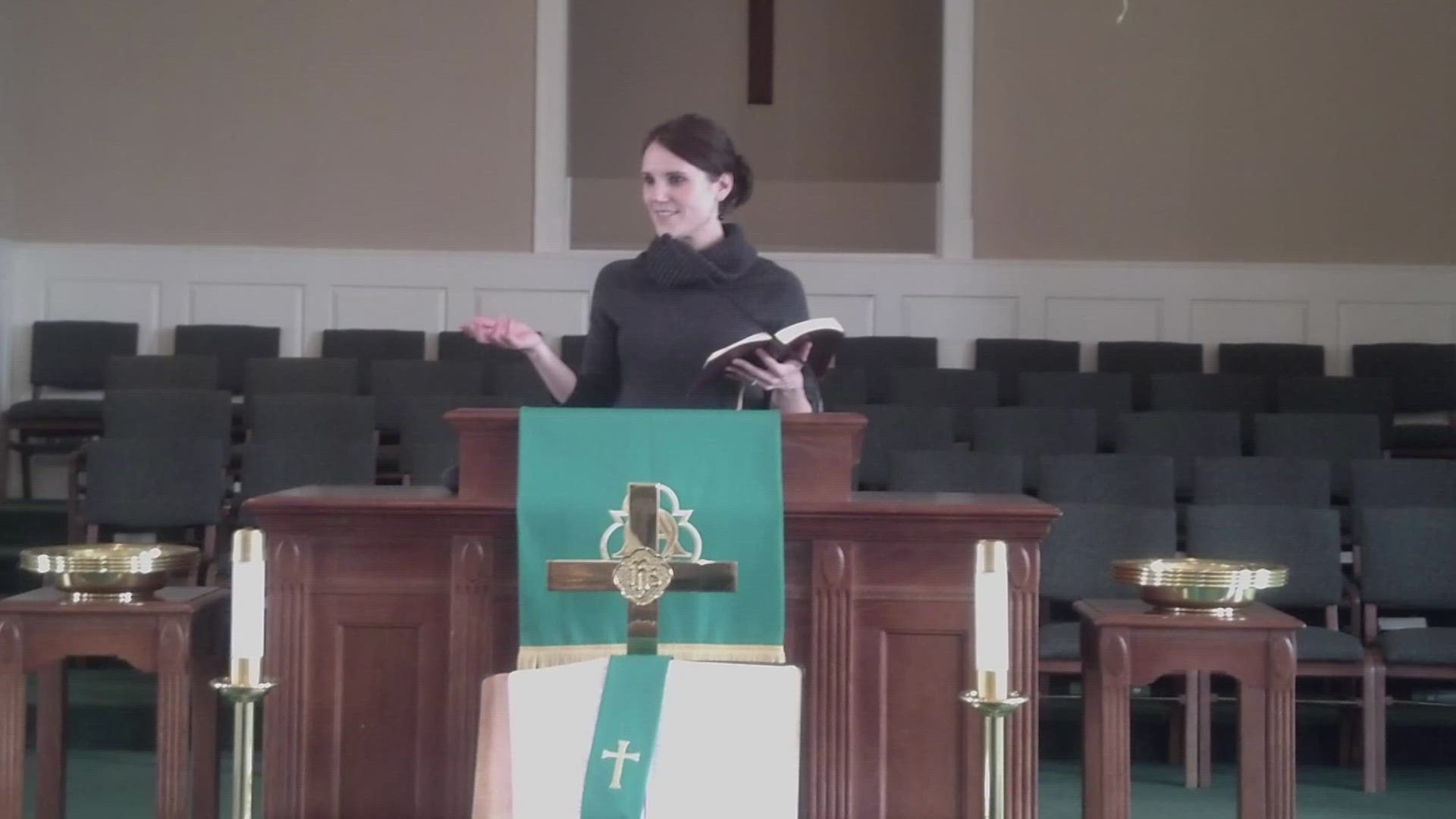A woman stands behind a large, dresser-sized, dark brown wood podium in a church. The podium features an elevated area for resting books. Draped on the front of the podium is a teal banner with a gold cross, and beneath it, another teal banner with a white cross. Two tall gold candlesticks with white candles are placed at the front. The woman, who is Caucasian with dark black hair pulled back, is wearing a gray sweater with a turtleneck-like top. She holds an open Bible in one hand and gestures with the other. Flanking the podium are two small side tables holding gold plates, and behind her are rows of gray chairs arranged in a choir-like formation. The church's tan walls have a white bottom half, completing the serene and sacred ambiance of the space.